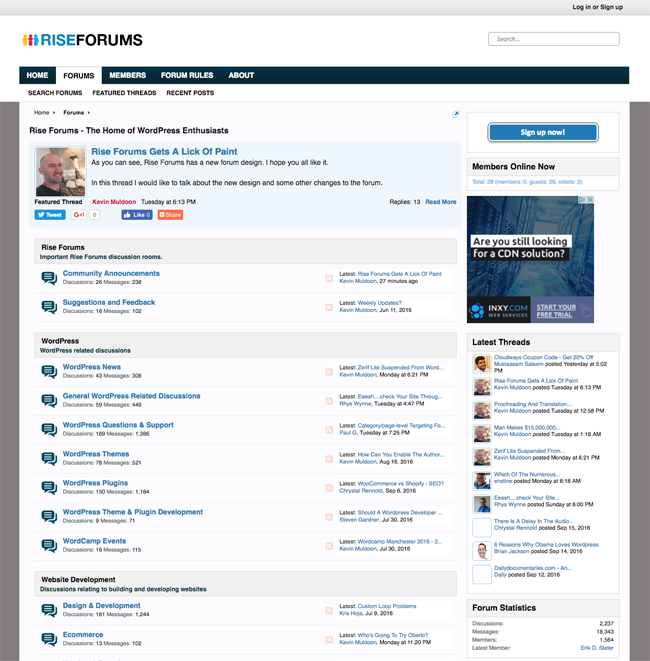Screenshot of the Rise Forums Website

The screenshot captures the user interface of a forums website named "Rise Forums." The top-left corner prominently displays the forum's logo, which features three small icons of people. The icons are colored differently: yellow on the left, red in the middle, and blue on the right. Next to the icon, the word "Rise" appears in blue, while "Forums" is written in black.

In the top-right corner of the screen, there is a search bar allowing users to search for content within the forum. Directly below the header, a black navigation bar features several tabs labeled Home, Forums, Members, Forum Rules, and About. The currently active tab is Forums, which stands out in white, while the others remain black.

The main content area below the navigation bar displays various forums in a list format. The first expanded section is titled "Rise Forums, the home of WordPress enthusiasts." This section includes a thumbnail image of a bald Caucasian man wearing a black t-shirt. The forum's highlighted topic is "Rise Forums Gets Lick of Paint," detailing the website's new design. The post reads, "As you can see, Rise Forums has a new forum design. I hope you like it. In this thread, I would like to talk about the new design and some other changes to the forum." Beneath this post, there are several social media sharing buttons, including options to tweet, like on Facebook, and an orange share button whose specific function is not immediately clear.

Continuing down the page, additional forums are listed under various categories: the "Rise Forums" section, which contains two articles, the "WordPress" section with multiple articles, and the "Website Development" section. On the right-hand side of the screen, there is an advertisement for Inksy.com and a "Latest Threads" section that highlights the newest discussions in the forum.